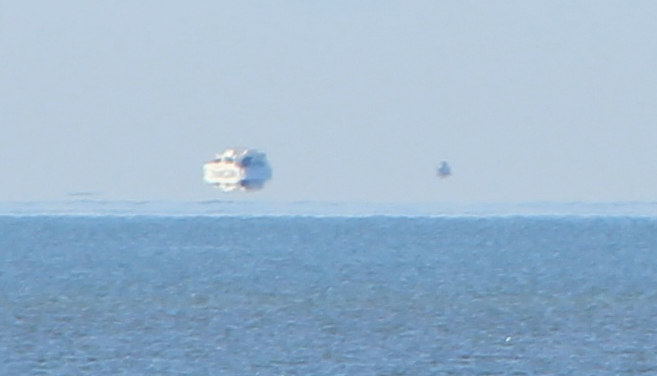In this intriguing image, we observe what appears to be a distant shot taken with a long-range zoom camera, capturing a scene that borders on the surreal. The main focus is a white boat positioned slightly to the left of center. Due to the photo's long-range nature, the boat looks as if it is floating above the gray-blue ocean, creating an unusual optical illusion. The boat's side is a long white rectangle, with a shorter white rectangle marking its front, although the details are indistinct because of the distance. This floating impression is only enhanced by the choppy, light blue water seen below, rippling in side-by-side patterns. In the upper half of the image, the sky mirrors the ocean with its own gray hue, blurring the lines between sea and sky. Additionally, on the right side of the center of the image lies a small, dark speck—possibly a bubble or a shadow—that adds to the enigmatic quality of the photo. The overall scene is puzzling and induces a sense of ambiguity, as if the objects are suspended in mid-air above the water.